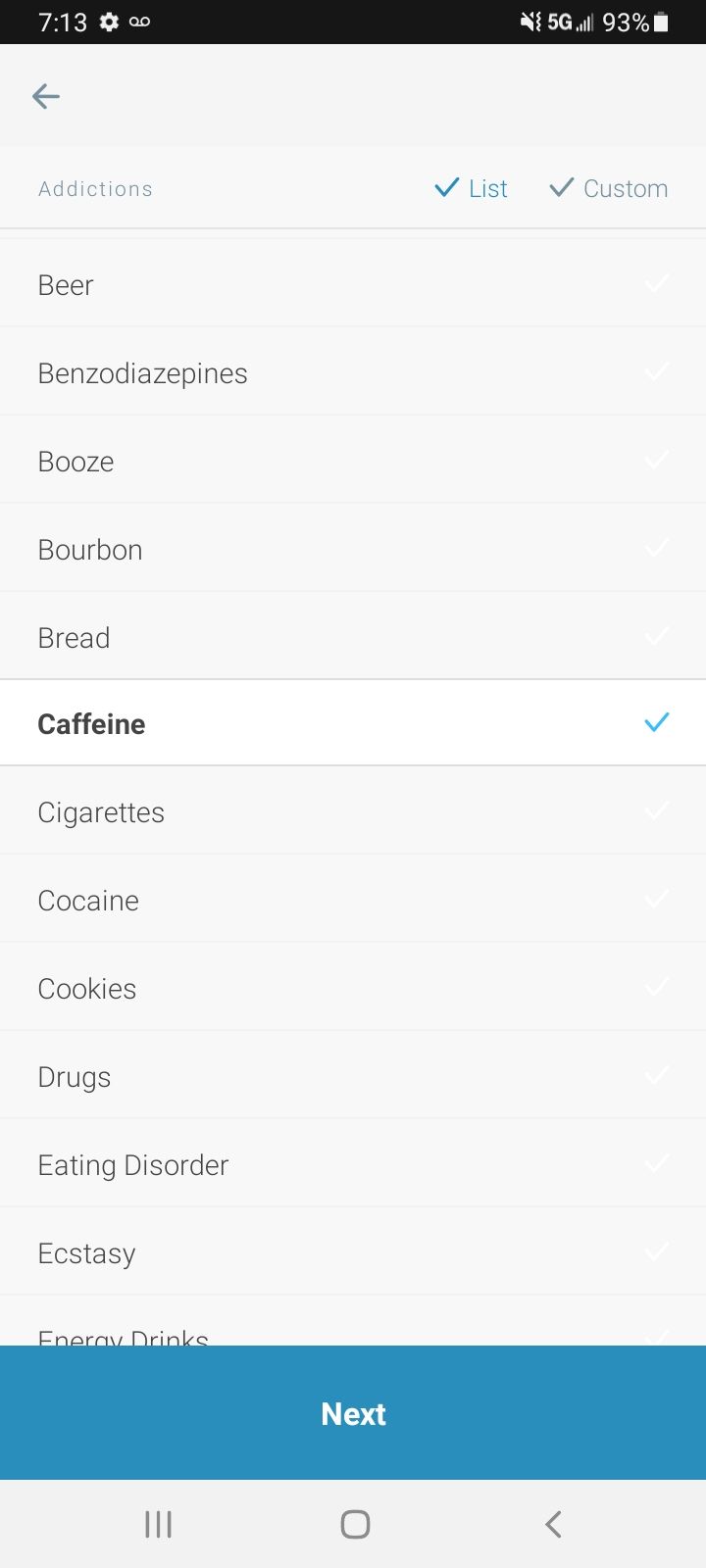This vertical rectangular image features a user interface likely from a mobile device. 

At the top, there is a black horizontal rectangular bar spanning from left to right. In the upper left corner of this bar, the time "7:13" is displayed in white font. Next to the time is a settings icon followed by another indistinct icon. On the far right of the bar, the battery level is shown as 93% with a nearly full white battery icon. 

The remainder of the image has an off-white background. Directly below the top bar, there is a left-pointing arrow. Beneath the arrow, the word "Addictions" is positioned on the left side. Adjacent to "Addictions," the word "List" is displayed in turquoise, preceded by a check mark. Following this, in gray text, is the word "Custom," also preceded by a check mark. Both "List" and "Custom" are on the same line.

Underneath "Addictions," a series of substances and behaviors are listed in unbolded black font: Beer, Benzodiazepines, Booze, Bourbon, Bread. Among these, "Caffeine" stands out as it is written in bolded black font within a crisp white rectangular area, contrasted against the off-white background, and marked with a turquoise check mark on the far right. The list continues in unbolded black font with: Cigarettes, Cocaine, Cookies, Drugs, Eating Disorder, Ecstasy, and Energy Drinks (which is slightly obscured).

Below this list, a blue horizontal rectangle intersects the image. This rectangle has the word "NEXT" in bolded white font.

At the bottom of the image, in the off-white background, are three vertical lines, a small circle bubble, and a "V" shape with the bottom pointing left, suggesting possible icons or menu options.